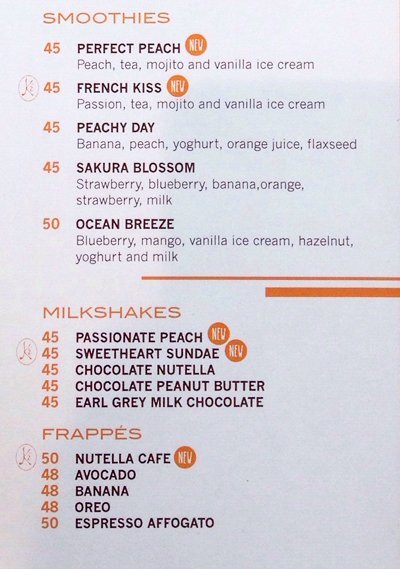This is a detailed menu showcasing a variety of smoothies, milkshakes, and frappes, all presented on a white background with black text and highlighted orange elements for the numbers, "new" indicators, and titles. The smoothie section includes new offerings such as Perfect Peach, which combines peach tea, mojito, and vanilla ice cream, priced at 45 (currency not specified). Also newly introduced is French Kiss, featuring passion tea, mojito, and vanilla ice cream, also priced at 45. Other smoothie options include Peachy Day (45) with banana, peach, yogurt, orange juice, and flaxseed, Sakura Blossom (45) with strawberry, blueberry, banana, orange, strawberry milk, and Ocean Breeze (50) combining blueberry, mango, vanilla ice cream, hazelnut, yogurt, and milk.

The milkshake section, all priced at 45, includes new additions such as Passionate Peach and Sweetheart Sundae, alongside existing flavors like Chocolate Nutella, Chocolate Peanut Butter, and Earl Grey Milk Chocolate.

In the frappes section, Nutella Cafe is a new item priced at 50. Additional options include Avocado (48), Banana (48), Oreo (48), and Espresso Affogato (50).